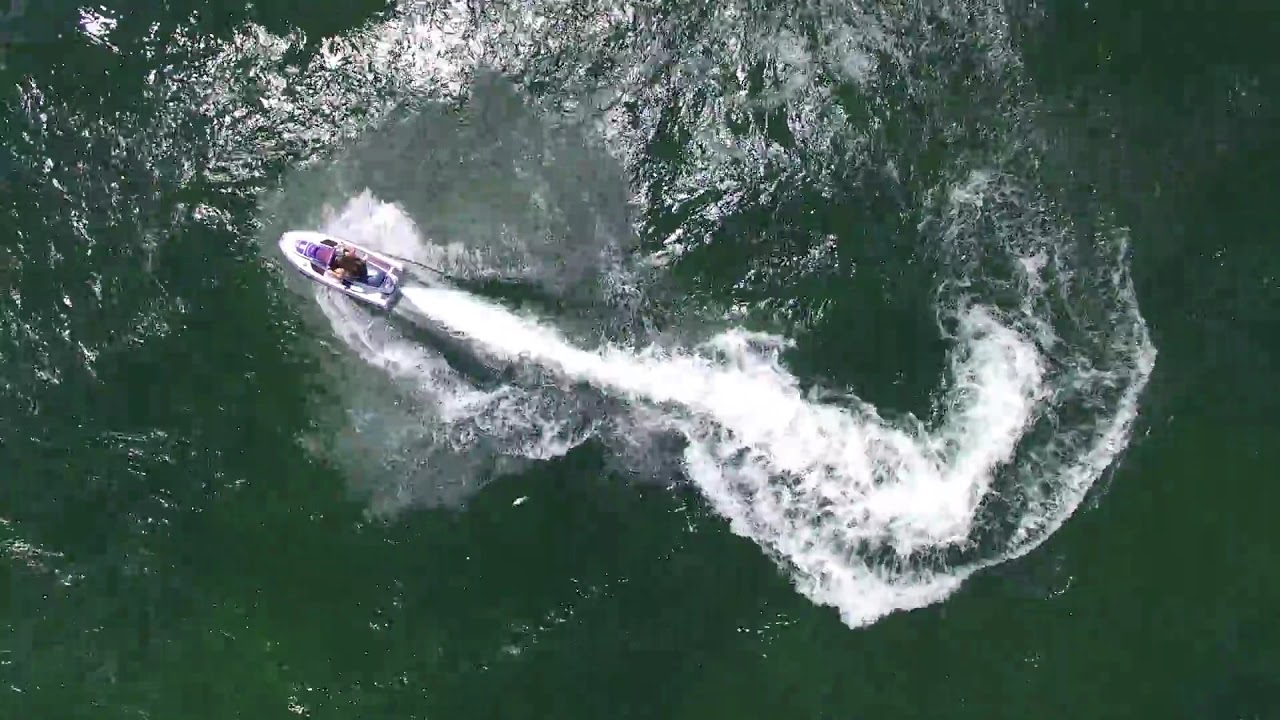The image is a direct aerial view, from an elevation of approximately 75 feet, looking straight down at a body of water with a deep forest green color. The camera captures a small, white motorboat traveling from the bottom right towards the top left of the frame. The boat, which appears to be able to seat around five people, has a distinct shape with a rectangular back tapering to a near-point at the front. The surface of the water is marked by sunlight glistening and reflecting, especially near the top edge. As the boat moves, it creates a large, foamy white wake that dramatically splits the water, adding a dynamic element to the image. The wake trails behind in a thick, streak-like formation, disturbingly the otherwise agitated green water. Some areas of the water further from the boat appear calmer and more still. The boat also features some darker colored accents, possibly purple, which add a subtle detail to its appearance.